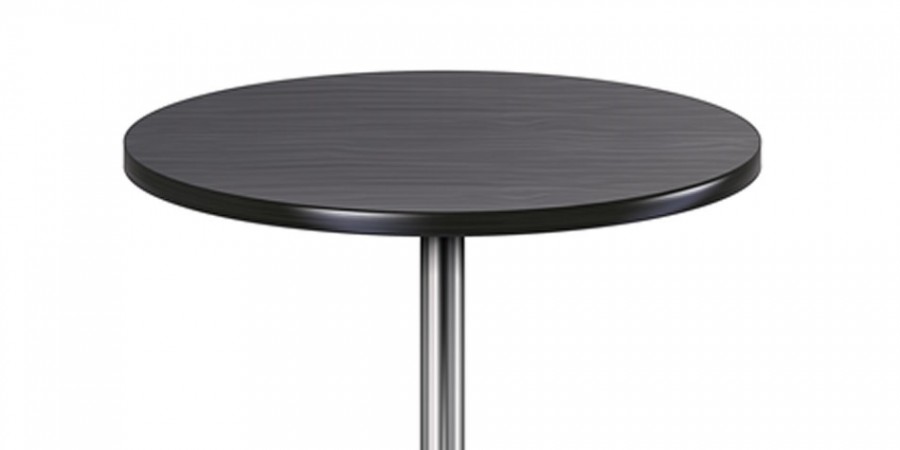This image presents a close-up, detailed view of a small, round tabletop mounted on a single, silver pole. The tabletop has a dark, almost black wood grain finish, with distinct horizontal lines visible across its surface, giving it a textured appearance. Encircling the edge of the tabletop is a shiny black trim, visually contrasting with the matte wood grain. The pole supporting the tabletop is silver, emerging from the center but not fully visible as the bottom part is cut off in the image. The backdrop is entirely white, devoid of any text, objects, or shadows, making the tabletop the sole focus of the composition.